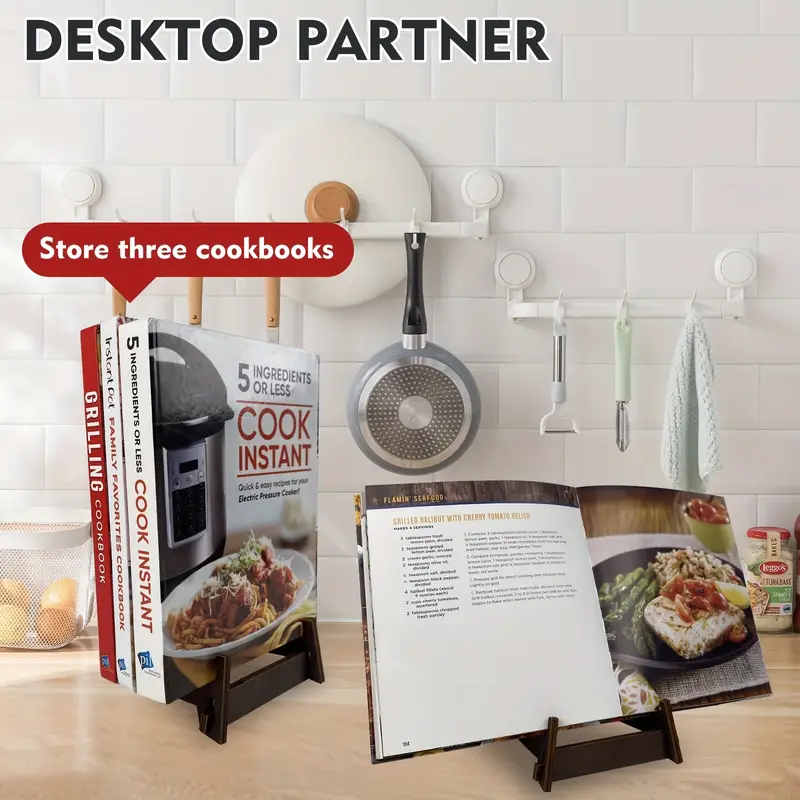The image portrays a bright kitchen scene featuring a versatile cookbook holder prominently labeled "Desktop Partner" in large font at the top left. The backdrop consists of a white-painted brick wall adorned with various kitchen utensils, including pots, pans, peelers, and a towel, all neatly hung from white hooks. The countertop, made of light birch-colored wood, supports a metal mesh basket filled with either fruit or eggs, positioned near the wall. 

Centered in the image is the main product—a dark brown, possibly mahogany, easel-style book holder. The stand is illustrated in two configurations: on the right, it holds an open cookbook displaying a recipe, and on the left, it supports three closed cookbooks, highlighted by a red text bubble that reads “store three cookbooks.” Sunlight filters in from a window on the left side, casting a warm glow over the scene, particularly illuminating the basket near the wall. The cohesive setup showcases both the functional and storage capabilities of the cookbook holder, making it a handy and stylish addition to any kitchen.